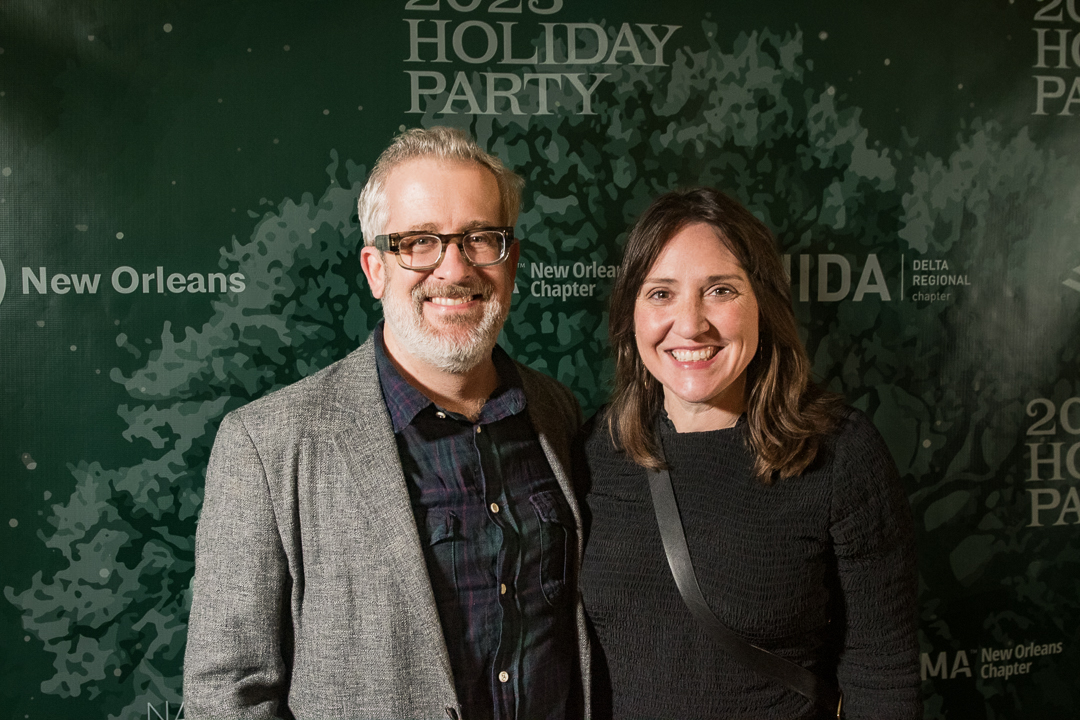The image captures a man and a woman standing side by side, both smiling warmly. The woman, positioned on the right, has shoulder-length brunette hair and is wearing a black long-sleeved top. She has a strap across her chest, likely from a purse or backpack. The man, positioned on the left, sports a gray suit jacket over a blue, purple, and green plaid collared shirt. He has short salt-and-pepper hair, a gray beard, and is wearing black glasses. The background features a predominantly green display with various texts including "Holiday Party," "New Orleans chapter," and "Delta Regional Chapter," along with logos and possibly a tree design. The two individuals stand at the center of the image, appearing to enjoy the festive atmosphere suggested by the backdrop.